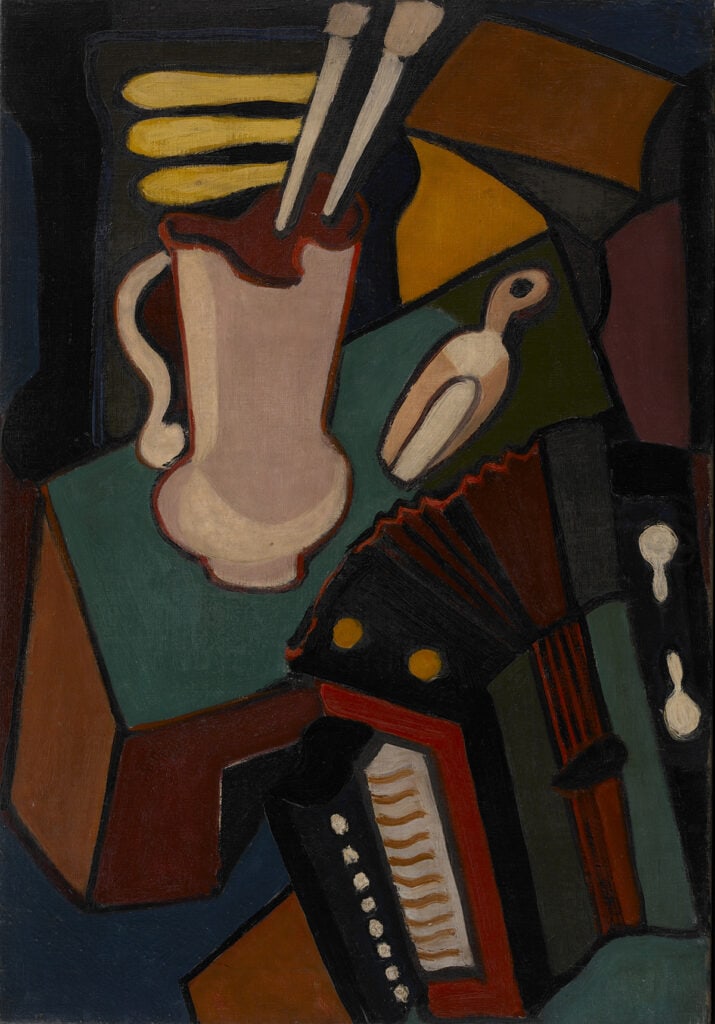This image features a contemporary, abstract painting titled "Still Life with an Accordion." The composition is infused with dark, moody colors like brown, dark teal, deep red, black, mustard yellow, gold, and creamy white, creating an atmospheric and almost somber tone. The painting, reminiscent of Picasso's style, presents a collection of identifiable yet disorganized objects depicted with a certain level of abstraction.

At the center of the piece, you can discern the shapes of an accordion, detailed enough to include its keys and buttons. Adjacent to it is a vase or cup-shaped object, depicted with orange outlines and a tannish base, containing what appear to be paintbrushes or straws. This container stands on a stool, which has a brown base and a green top. Additionally, the painting includes a table and some kind of scoop, contributing to the overall cluttered arrangement of objects.

The lighting in the painting suggests a setting where the light source is behind the artist, casting reflections from the left side and creating a depth that emphasizes the moody color palette. The abstract nature of the piece leaves some details unclear, adding to its enigmatic quality and enhancing its contemporary style.